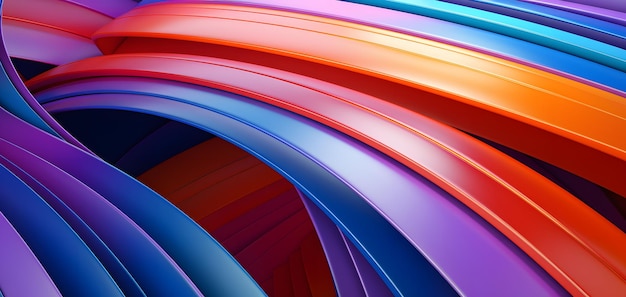The image features an array of multicolored, thick bands, predominantly in shades of blue, purple, red, yellow, orange, and turquoise. In the lower left-hand corner, blue and purple bands dominate. These bands, which resemble flat plastic tubes, are either straight or bent and stretch diagonally from the upper left to the bottom right of the rectangular, horizontal photo. The bands are bisected by a distinct groove and lie against a brown, wooden surface visible between the two groups of bands. The picture is vividly colorful and entirely composed of these bent and straight stripes, with no text or additional elements present.